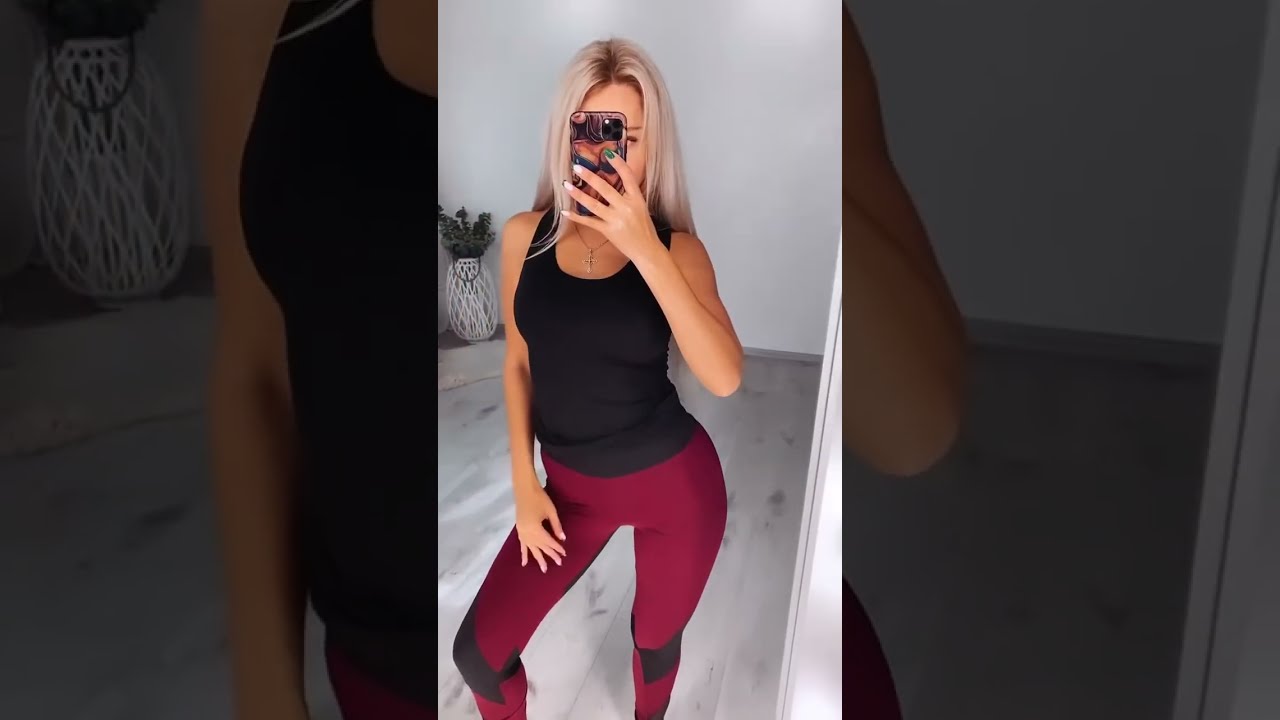The image features a Caucasian woman inside a bright, white-wood-floored room, taking a selfie while facing a mirror. Her long, dirty blonde hair flows down past her shoulders with a darker brownish hue near the roots. Holding an iPhone with a colorful case in her left hand, she poses with the phone obscuring her face. Her fingernails are painted in various colors. She is dressed in a form-fitting black tank top and striking burgundy workout leggings with black knee patches. A subtle necklace adorns her neck, complementing her casual yet stylish look. In the background on the left, a large floor vase filled with indistinct, possibly green vegetation adds an element of decoration to the indoor setting, which is bathed in natural daylight. The overall image composition has a horizontal orientation, with the detailed central vertical picture of the woman providing a focal point. Cementing the image's modern aesthetic, it also evokes a sense of social media presence similar to platforms such as TikTok or Instagram.